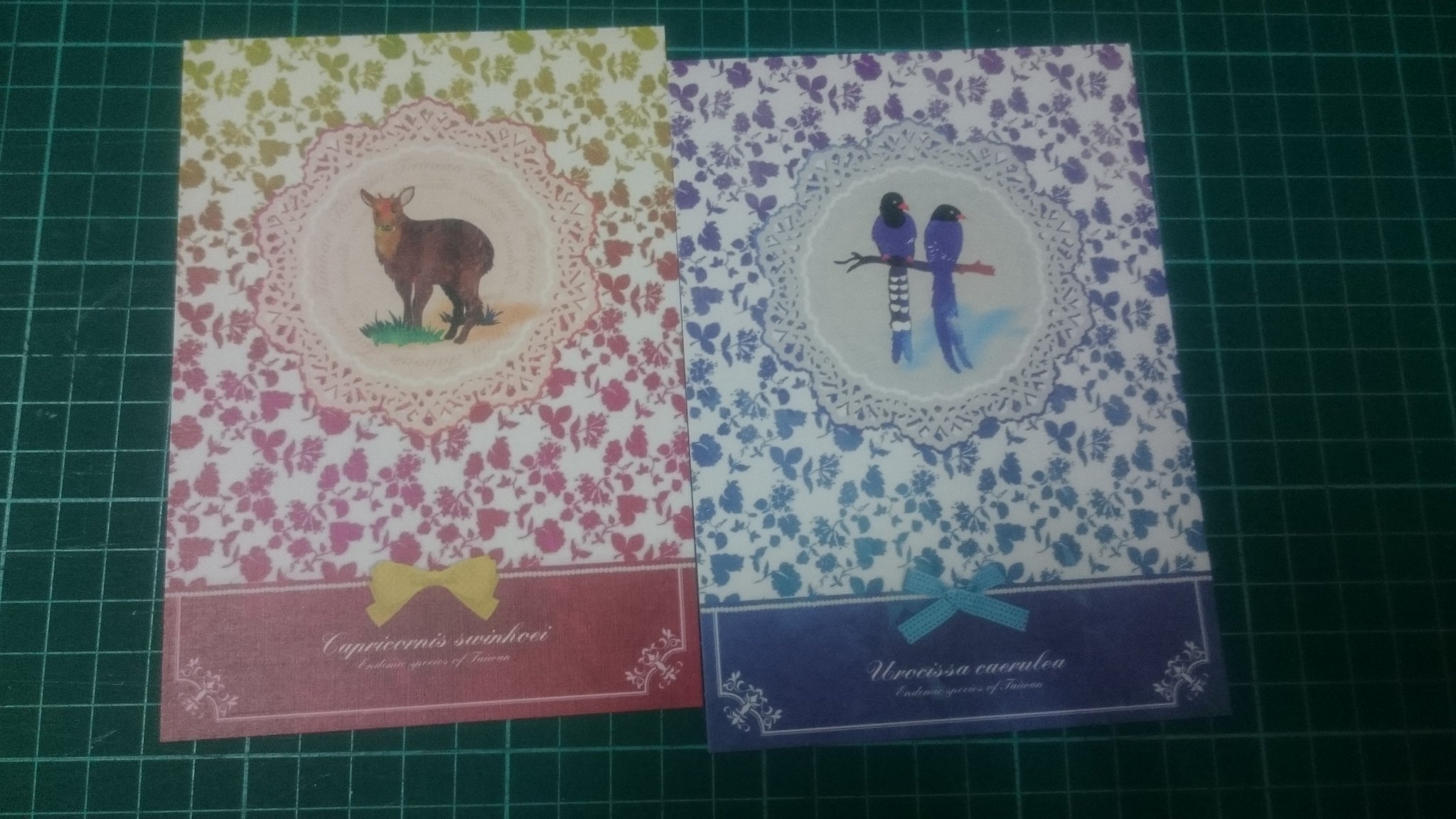This image displays two intricately packaged tablecloths, each distinct in color and design. The first tablecloth, with its packaging, is predominantly green on the top and transitions to a pinkish-red on the bottom. Adorning this tablecloth is a doily featuring a detailed illustration of a deer standing on brown ground, surrounded by a patch of grass. The doily itself is tinged with a reddish-pink hue, complementing the lower part of the packaging, which is highlighted with a gold bow.

The second tablecloth is presented in a similarly ornate fashion. It comes in blue packaging, distinguished by a white doily in the center. The doily depicts two blue birds with black heads perched on a twig, their notably long tails adding elegance to the design. Beneath the birds, there is a subtle hint of blue ground. This tablecloth is wrapped in packaging that has a blue strip at the bottom and is adorned with a blue bow.

Both of these tablecloths, encased in their refined packages, are set against a green background composed of various square patterns. This layout enhances the vibrancy and detailed presentation of each tablecloth's packaging.